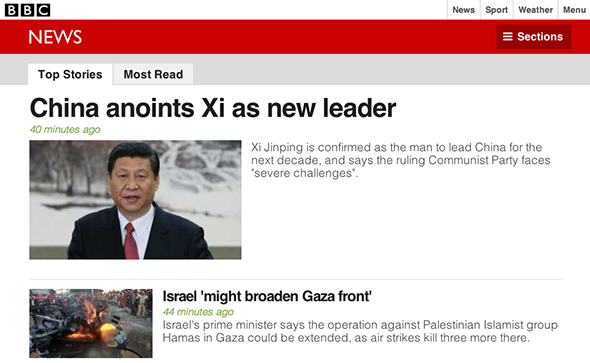The image displays a webpage from the BBC News site. In the top left corner, the BBC logo is visible, while the top right corner features the words "News," followed by the numbers "4" and "1," along with the "Menu" option. A prominent red bar stretches across the top, containing the word "News." Beneath it, there is a section labeled "Sections," followed by a grey area.

Below this, there are two tabs: "Top Stories" and "Most Read." The main headline reads "China Annoyance," with a subheading indicating that "Xi Jinping is confirmed as the man to lead China for the next decade." This headline is accompanied by a timestamp of "40 minutes ago" and a smaller picture of Xi Jinping wearing a tie. The text further elaborates that "the ruling Communist Party faces severe challenges."

Additionally, towards the bottom left of the image, another story is partially visible, headlined "Israel Playing Proud in Gaza Front," timestamped "41 minutes ago." The brief summary notes that "Israel's Prime Minister says the operation against Palestinian Islamist group Hamas in Gaza could be extended as airstrikes have killed three more individuals there."

The background comprises various text elements, predominantly in white and red, contributing to the detailed and information-rich presentation of the news on the BBC webpage.